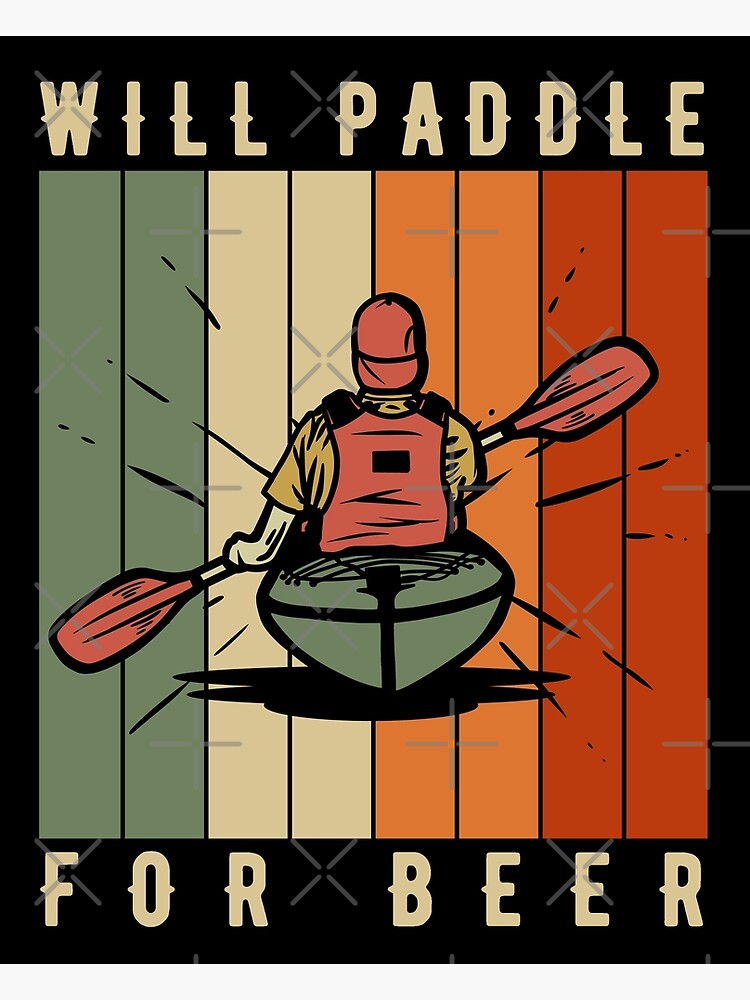The poster is a visually striking, vertical rectangular frame primarily featuring a vibrant and colorful digital graphic. At the very top of the poster, against a black background, the phrase "WILL PADDLE" is boldly displayed in uppercase white font. At the very bottom, it reads "FOR BEER" in the same style, framing the central image which captures the majority of the space.

The central image itself is a square with a vivid, horizontally-striped background composed of eight distinct colored stripes: two forest green, two olive green, two orange, and two dark red. Sitting against this backdrop is the figure of a man viewed from behind. He appears to be paddling, seated in a green kayak. The man is wearing a yellow t-shirt, an orange flotation vest, and a red cap turned backward. His hands grip a paddle with a white shaft and red blades at both ends, resting across his lap. The man, who seems to have a Caucasian complexion, is depicted in an illustrative or animated style, suggesting a promotional or whimsical intent, likely suitable for a bar or cantina setting.